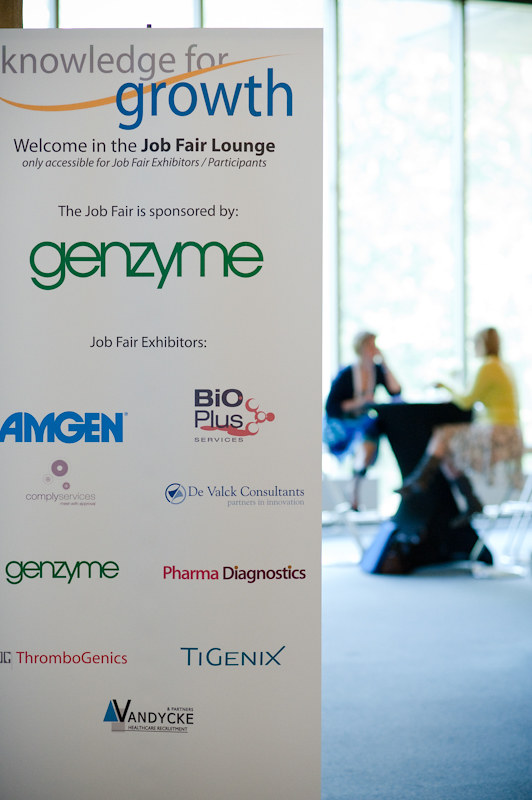The image depicts a professional meeting space with a significant focus on a job fair event. In the background, two women in business attire are seated at a table, engaged in conversation, and perched on high chairs against a backdrop of impressively tall windows that allow ample natural light into the room. In the foreground, a prominently positioned banner, sharply in focus, reads: "Knowledge for Growth. Welcome to the Job Fair Lounge, only accessible for job fair exhibitors and participants." The event is sponsored by GemZon and features exhibitors such as AmGem, BioPlus, Devout Consultants, Pharma Diagnostics, Tigenics, Van Dyke, Thrombogenics, Genzyme, and Comply Services. The overall setting conjures a professional and collaborative atmosphere, ideal for networking and job opportunities.